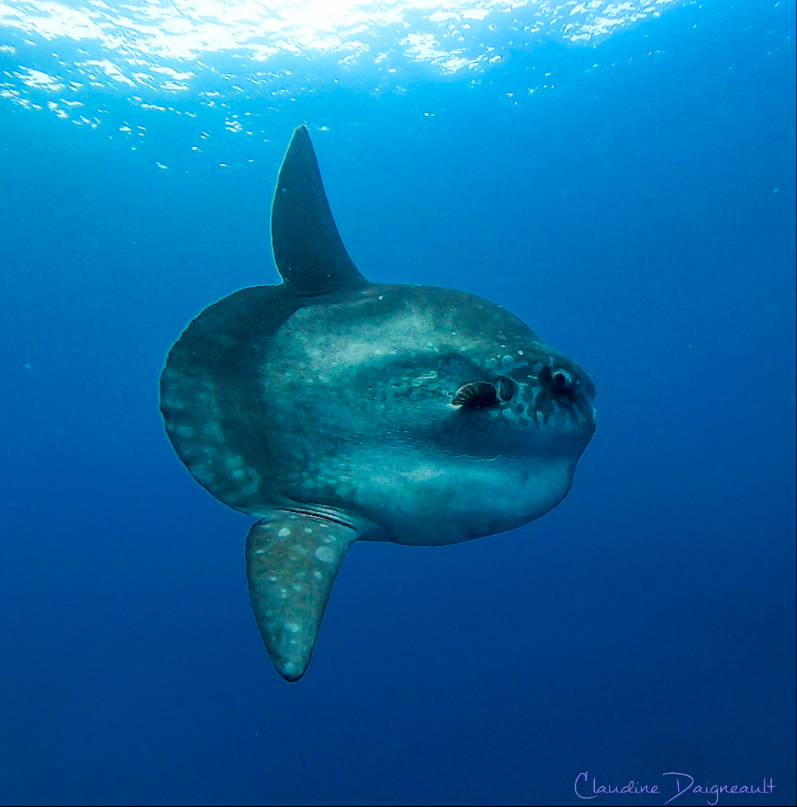This is an actual photograph taken by Claudine Daignault Dorbenacht of an underwater scene featuring a distinctive fish. The fish, somewhat resembling a puffer fish or possibly a small shark, is notably thick and compact in an oval shape. Its body displays a unique blend of dark turquoise with black and darker splotches. It has fins that extend both upward and downward, akin to arm fins on either side, and a tail that flares out uniformly, resembling the tail feathers of a chicken. The background is a dark blue, with light filtering through the water’s surface, casting white reflections and creating gentle splashes near the top of the photo. This suggests the photo was taken relatively close to the surface, possibly while Claudine was scuba diving. Bubbles and the underwater lighting contribute to the serene yet vivid depiction of this intriguing aquatic scene.